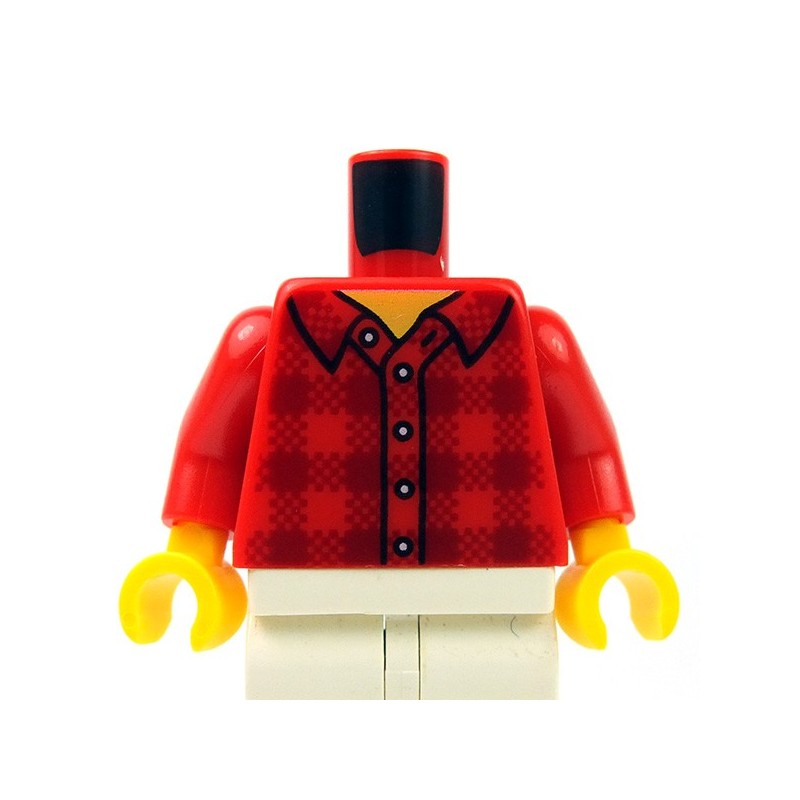The image depicts a professional-quality photograph of a headless Lego figure centered against a stark white backdrop. The Lego body is adorned in a red, button-down shirt featuring a collar, white buttons (with the top button undone), and black detailing, giving the impression of plaid. Beneath the shirt, the Lego figure wears white pants. The arms are red and seamlessly extend from the torso, ending in yellow, curved appendages that are typical of Lego figures' hands. The figure's missing head reveals a red cylindrical protrusion, standard for attaching interchangeable Lego heads. The overall composition is minimalistic, with no props or text, emphasizing the sharp, well-lit details of the Lego piece.